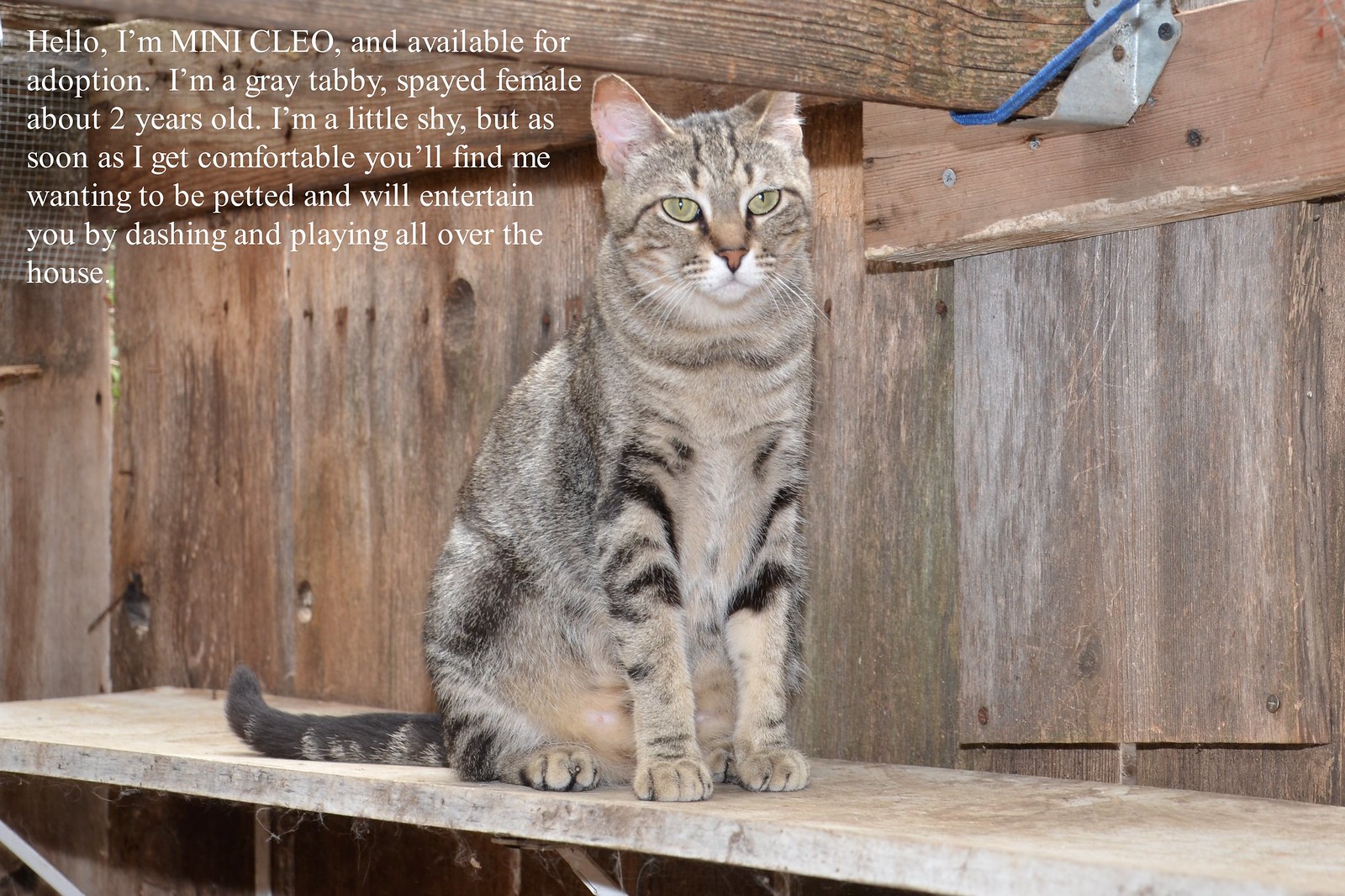In this detailed image up for adoption, we see a striking gray tabby cat named Mini Cleo. She's sitting attentively on a thin white, possibly marble counter that contrasts with the rough, unfinished brown wood behind her and above her head. Mini Cleo has piercing green eyes and distinctive black stripes, especially noticeable on her front limbs. Positioned with her front legs straight and her back legs folded beneath her, she looks slightly to the side of the camera, exuding a calm but curious demeanor.

The background features a rough, wooden wall with visible paneling, exposed screws, and what appears to be a blue binding on one of the upper wooden supports. On the upper left of the image, white text introduces Mini Cleo and provides more information about her: "Hello, I'm Mini Cleo and available for adoption. I'm a gray tabby spayed female, about two years old. I'm a little shy, but as soon as I get comfortable, you'll find me wanting to be petted and will entertain you by dashing and playing all over the house." This text snippet not only gives insight into Mini Cleo's personality but also emphasizes her readiness to find a loving home. The entire scene is beautifully rustic, drawing all focus to the solitary cat standing out against her wooden surroundings.